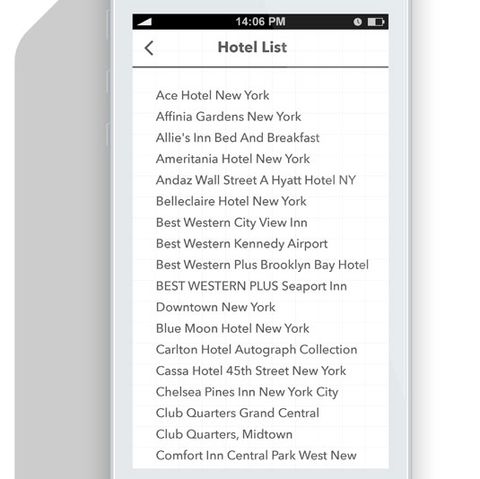This rectangular image features a list of hotels on a white background with text. A subtle gray border runs along the left side of the image. At the top, a black bar displays the time "14:06 p.m." with a clock icon on the left side and a battery icon on the right. Below this bar, the heading "Hotel List" is displayed, followed by a comprehensive list of hotel names, each formatted neatly in rows.

The list includes:
1. Ace Hotel New York
2. Athena Gardens New York
3. Alley's Inn Bed and Breakfast
4. Merita Hotel New York
5. Andy's
6. Wall Street
7. A Hyatt Hotel NY
8. Belcler Hotel New York
9. Best Western City View Inn
10. Best Western Kennedy Airport
11. Best Western Plus Brooklyn Bay Hotel
12. Best Western Plus Seaport Inn Downtown New York
13. Blue Moon Hotel New York
14. Carleton Hotel Autograph Collection
15. Casa Hotel 45th Street New York
16. Chelsea Pines Inn New York City
17. Club Quarters Grand Central
18. Club Quarters Midtown
19. Comfort Inn Central Park West New York

A gray border encircles the image’s content, extending across the top, left, right, and bottom sides. Additionally, a line separates the heading "Hotel List" from the subsequent listing of hotel names, enhancing the visual organization of the image.